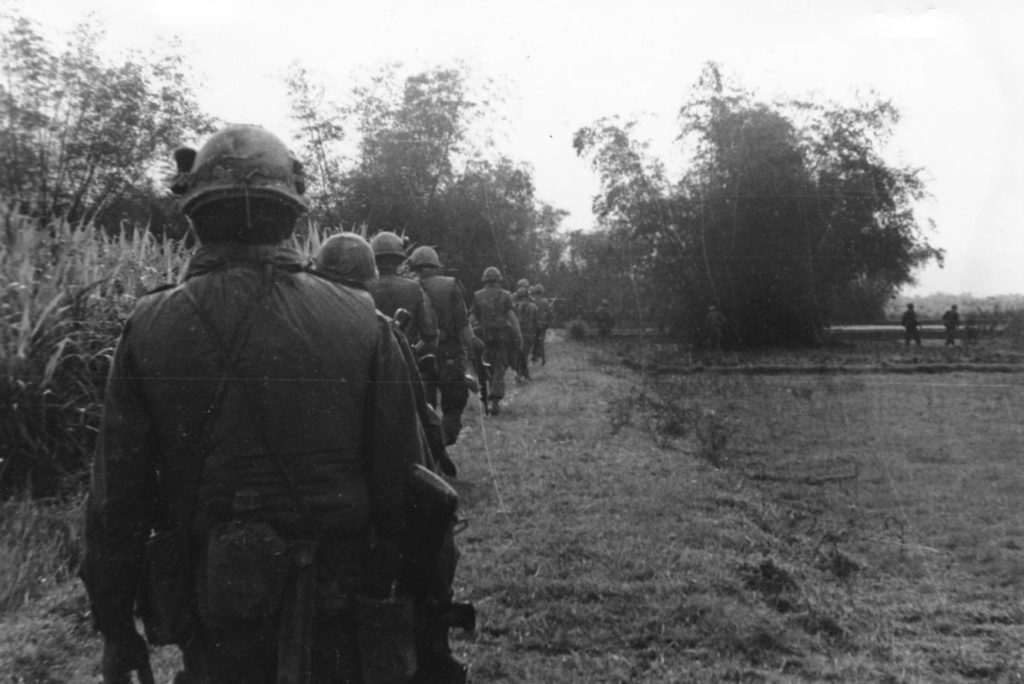This black and white photograph captures a poignant scene potentially from the Vietnam War era, depicting a line of soldiers walking single file along a berm. The soldiers, dressed in combat uniforms and wearing helmets, march with their rifles down. The focus is on the back of the last soldier in line, who is carrying a large gun in his right hand and a canteen attached to his belt. To their left, tall sedge grasses and some trees are visible, while to their right, two shadowy figures stand amidst a field of short grass, framed by a distant line of trees and possibly a body of water. The bright white sky adds to the starkness of the scene, evoking a sense of historic solemnity.